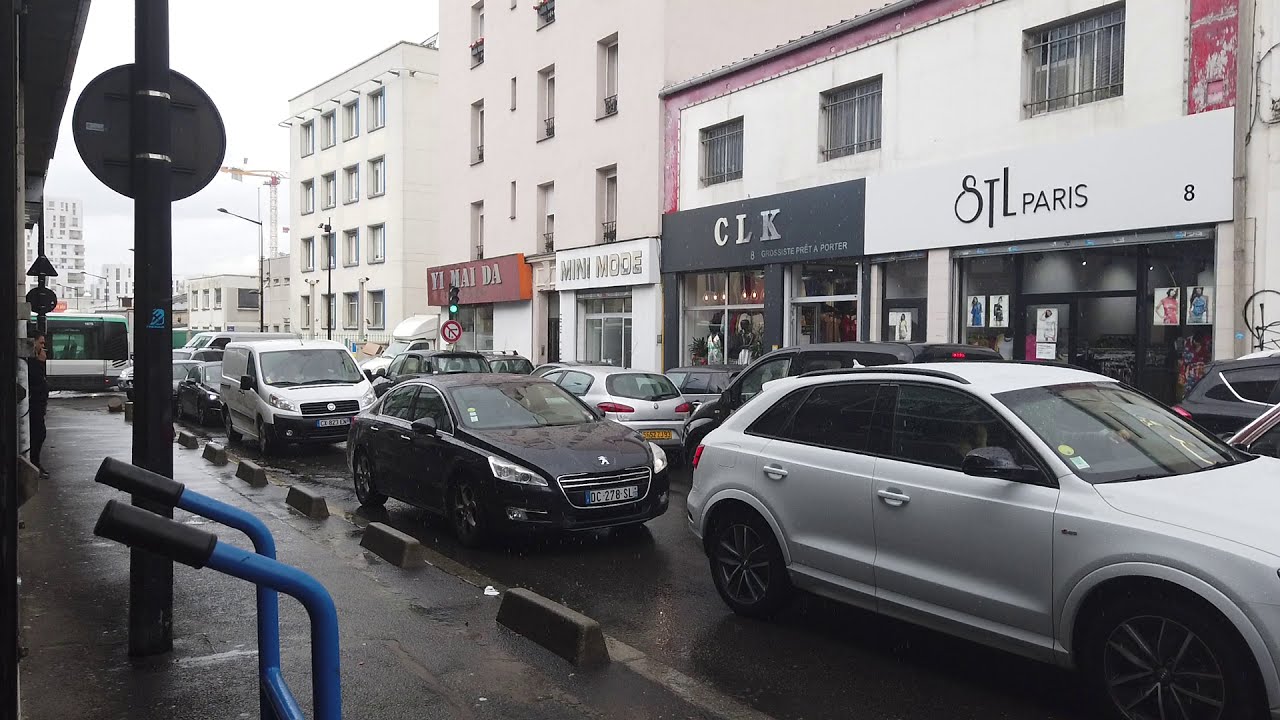The image captures a narrow, congested city street, possibly in Paris, lined with rectangular buildings featuring rectangular windows, some with bars on top. Storefronts are visible, one marked with "TL Paris" and another with "CLK", along with other unreadable signs. Vehicles, predominantly white, black, and gray sedans with black wheels and rims, are parked along both sides of the street, creating a busy atmosphere. Toward the bottom left corner, the blue handles and grips of a hand truck are visible. A black signpost with a circular black sign is present in the upper left corner. In the background, a bus can be seen on the left, and a traffic light with a green signal is observable under the overcast sky.